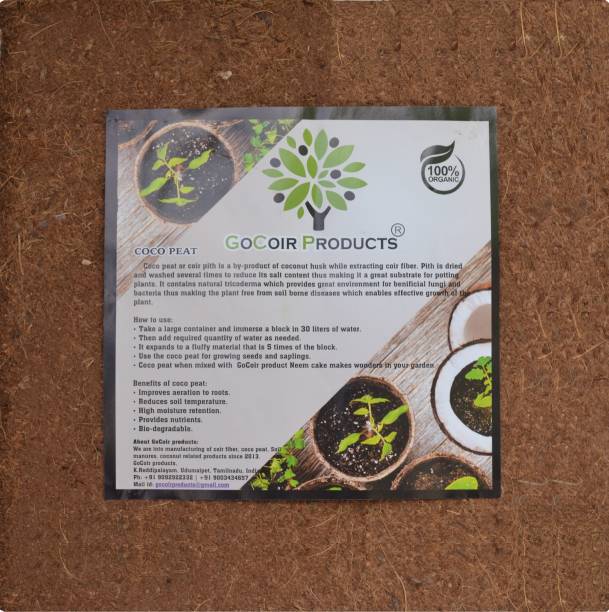The image is an advertisement for 100% organic Go Coir products displayed against a brown background. At the top left and bottom right corners, there are little potted plants with sprouts just starting to bloom. The main section occupies the middle of the image, featuring a gray square with a black border, containing key information about 'Cocoa Pete,' a byproduct of coconut husk rich in beneficial fungi and bacteria. The top right corner showcases a circular emblem with the text "100% organic" encircled by a leaf design. To the left of this is a stylized black tree with green leaves and black circles, possibly representing fruit. Next to the tree, the text "Go Coir Products" is written in black and green lettering. 'Cocoa Pete,' written in bold black letters, indicates instructions for immersing a block in 30 liters of water to expand it into a fluffy material, suitable for seeds and saplings. Additionally, mixing Cocoa Pete with Go Coir's neem cake enhances garden results. Benefits listed include improved root aeration, reduced soil temperature, high moisture retention, nutrient provision, and biodegradability. The bottom of the image mentions the company's contact information and website, though details aren't fully legible.